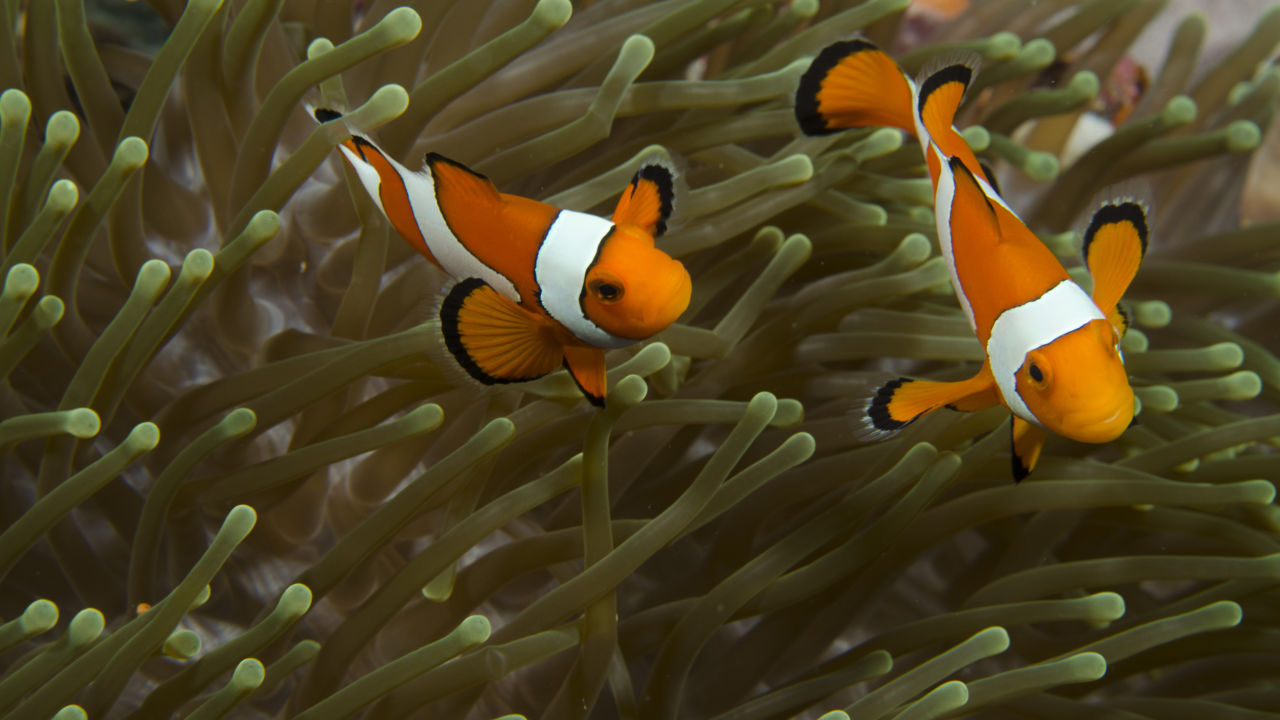This detailed underwater photograph captures two vibrant clownfish swimming close together among the flowing green tentacles of a sea anemone. The scene is set near the ocean floor with the light green anemone creating a lush backdrop, its delicate fronds gently swaying in the water. Both clownfish are bright orange, adorned with two thick white stripes encircling their bodies, and trimmed with black along the edges of their fins. The fish on the right faces the viewer, its tail pointing upwards, while the slightly smaller fish on the left appears in profile. This realistic image, in landscape orientation, vividly portrays the essence of an underwater habitat.